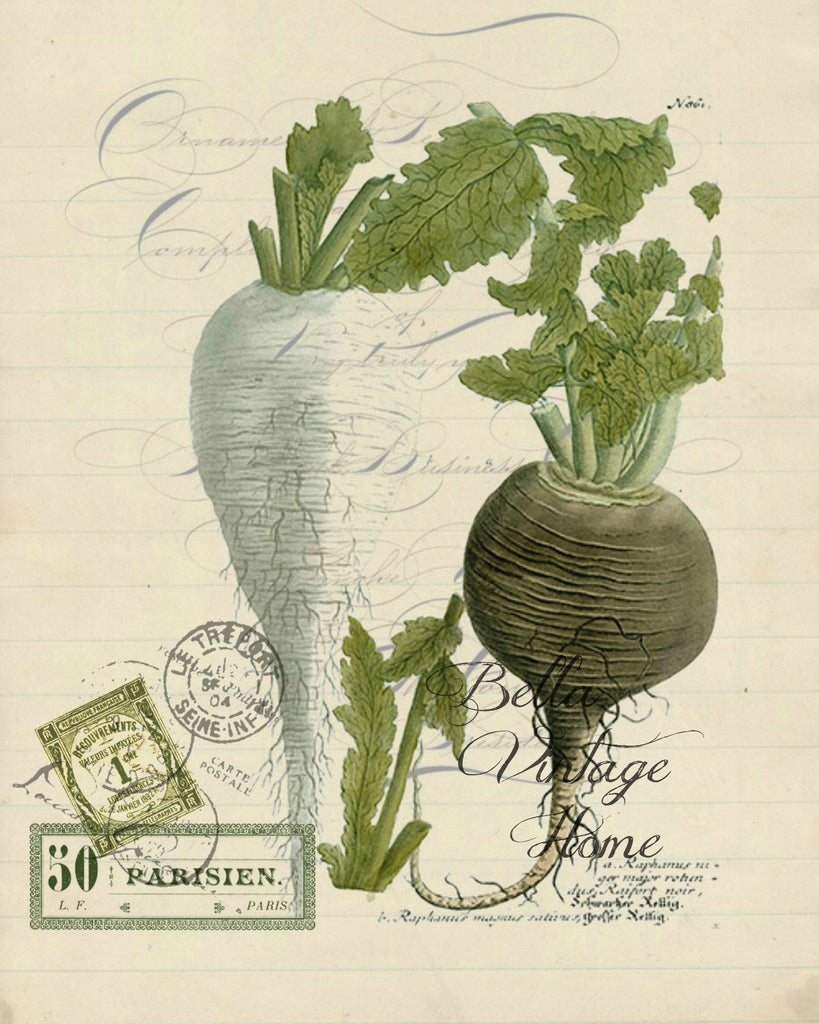This antique-style poster features a highly detailed illustration of two radishes at its center, rendered in a monochromatic scheme with green stalks and leaves extending from their tops. The radish on the left is large and white, while the radish on the right is somewhat more cylindrical with an olive-brown hue and a longer end. The background of the poster is cream-colored, adorned with horizontal lines resembling those of school paper, and includes cursive calligraphy strokes that enhance its vintage aesthetic.

In the foreground, text in cursive script reads "Bella Vintage Home," contributing to the old-fashioned appeal, while the bottom left corner features three antique-looking stamps reminiscent of postal stamps. Additional text, "50 Parisian," and other ineligible script are also visible, enhancing the impression that this piece might serve as decor in a restaurant or a vintage-themed kitchen. The careful interplay of text and image, combined with the overall aged appearance, gives this piece an air of nostalgic charm.